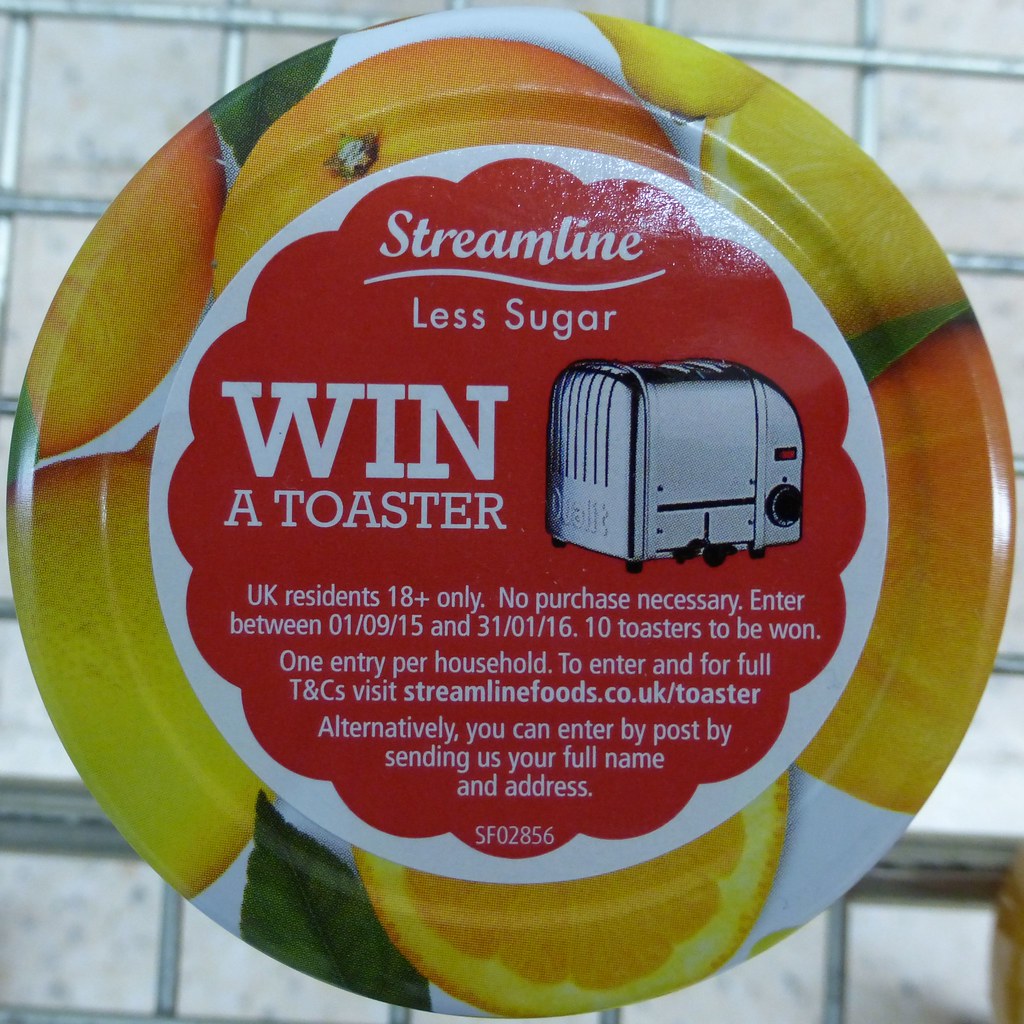The image features a detailed close-up of a promotional food label designed to look like a jar lid, likely for a jar of preserves or jam. The lid is predominantly red with a floral design, accented by a white rim. Surrounding the edge of the lid are images of whole and halved oranges, adding a vibrant touch of orange and green to the overall color scheme. Centered on the lid is a depiction of a silver toaster, emphasizing the promotional aspect of the label. The text, all in white, prominently reads "Streamline Less Sugar," followed by "Win a Toaster." Further information includes the eligibility requirements for UK residents aged 18 and over, stating no purchase is necessary. The entry period is from January 9, 2015, to January 31, 2016, with 10 toasters available to be won, one entry per household. Instructions for entering the contest direct participants to visit streamlinefoods.co.uk/toaster or submit their full name and address by post. The label also includes the reference code SF02856 at the very bottom.